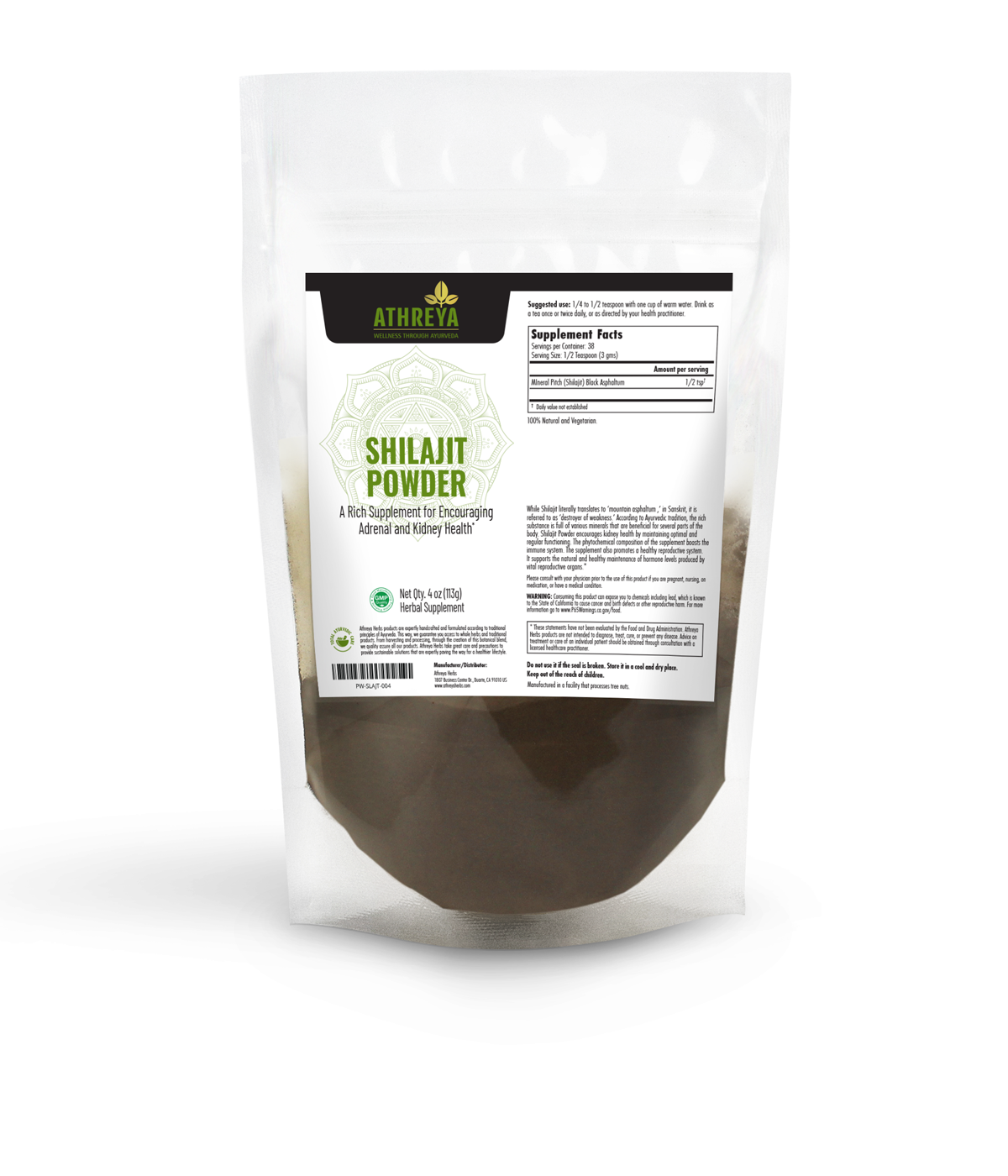A detailed, colored indoor photograph depicts a clear, Ziploc-style plastic bag, approximately 3 inches wide and 6 inches tall, filled with a brown powder. The bag displays a white food label embellished on the right side with black lettering and a green shield on the left that reads "SHILAJIT POWDER" in capital letters. Beneath this, in smaller print, it states: "A rich supplement for encouraging adrenal and kidney health." The label extends towards the bottom with finer print that isn't legible, likely detailing the contents and additional product information. Additionally, the label features the logo "Athreya" at the top left corner. The powder inside the bag appears dark brown at the bottom, transitioning to a lighter tan near the top. The backdrop of the image is a stark white, highlighting the clear, translucent bag and its contents.